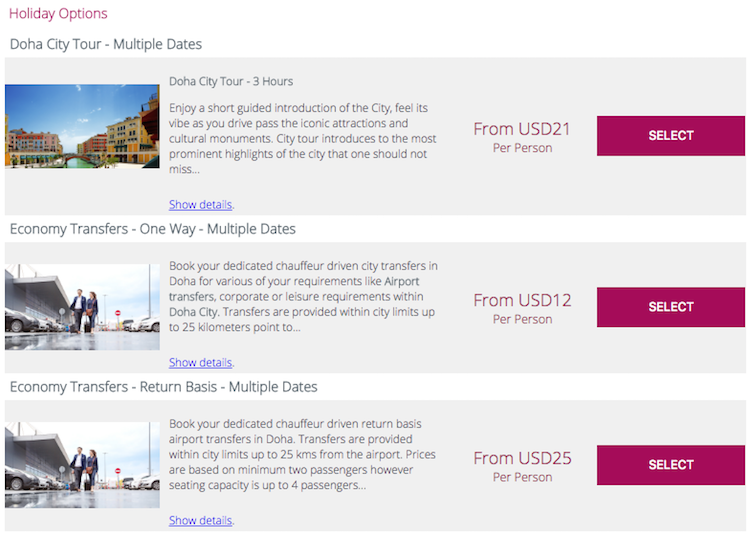Explore holiday destinations and their prices with this detailed guide. 

**Option One: Doha City Tower**
- **Multiple Dates Available**
- **Tour Length:** Three hours
- **Price:** Starting from $21 per person

Indulge in a short, guided tour of Doha's iconic landmarks and cultural treasures. This tour offers a comprehensive introduction to the city's vibrant atmosphere, allowing you to experience its renowned attractions and significant monuments. The City Tower tour highlights the most essential sights that every visitor should see.

**Additional Options:**

- **Economic Transfers (One-way):**
  - **Multiple Dates Available**
  - **Price:** Starting from $12 per person

- **Economic Transfers (Return):**
  - **Multiple Dates Available**
  - **Price:** Starting from $25 per person

These economic transfer options provide affordable and convenient transportation to ensure you make the most out of your visit to Doha.